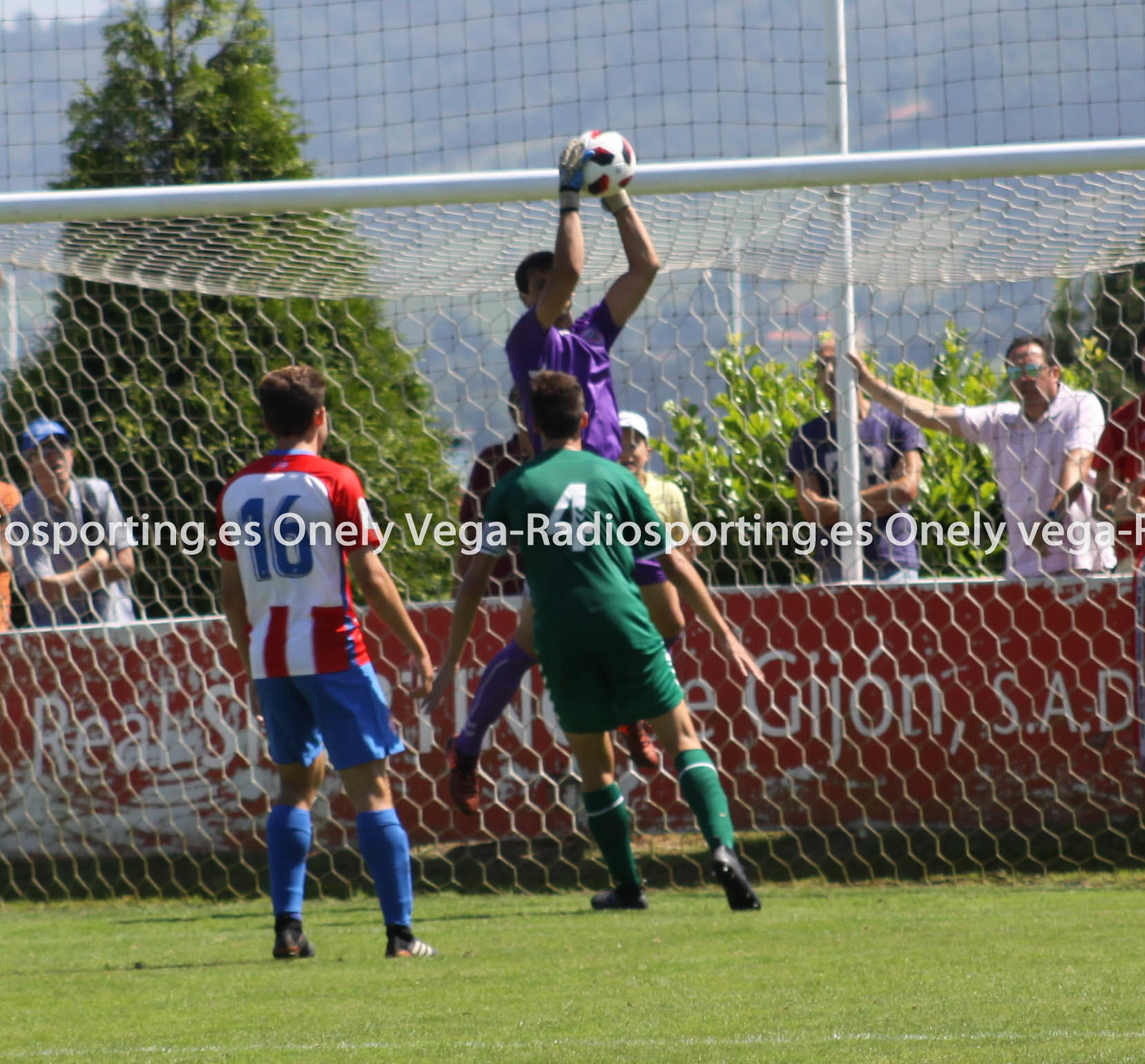This outdoor photograph captures a dynamic moment in a soccer game during daylight. At the center, a dark-skinned goalie, dressed in a purple short-sleeve jersey and shorts, is airborne, having just caught a white soccer ball with red and black stripes in front of the goal net. His short, dark hair is partially obscured by his arms. To the left, player number 16 has his back to the camera, identifiable by his short brown hair and red, white, and blue jersey, paired with blue shorts and socks. To the right, player number 4, wearing an all-green outfit with matching green knee-high socks and black cleats, faces the goalie. Both players are of Caucasian descent. In the background, spectators stand behind a concrete border painted red with various white inscriptions, including "Real" and "Gijon S.A.D." To the left of the scene, a man in a blue hat folds his arms, while another in a purple shirt and one in a white shirt with sunglasses cheer. Beyond them, lush green trees and bushes frame the scene under a clear blue sky. Spanning the concrete border, white text reads "osporting.es."